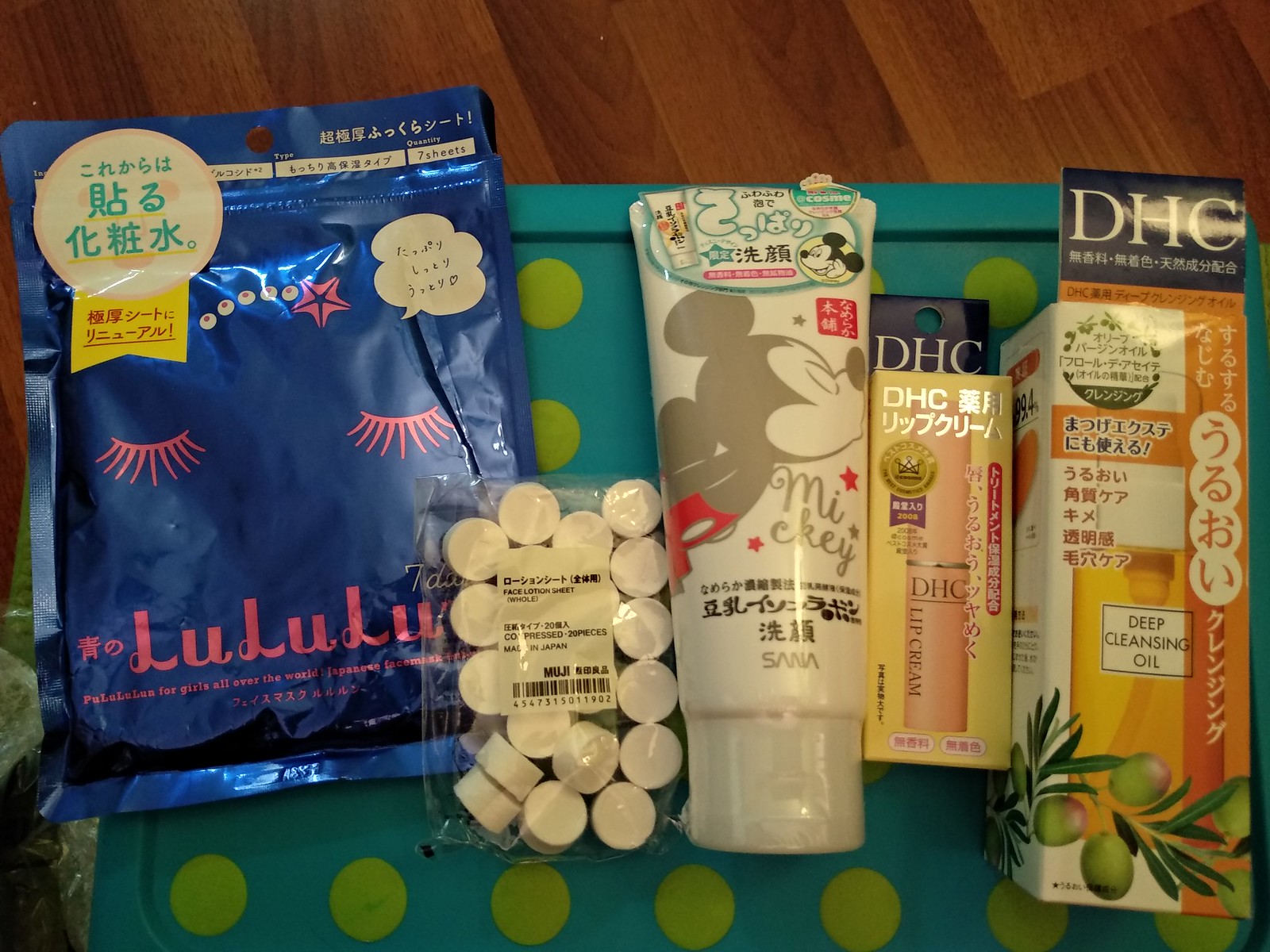This image showcases an array of health and beauty aid products, all distinctly featuring Asian character scripts, though it's unclear whether they are Korean, Japanese, or Chinese. The various products are meticulously arranged on what appears to be a turquoise square plastic surface, possibly a lid, adorned with neatly aligned green dots forming rows.

Starting from the left, there is a bright blue, square-shaped bag with a tear-off top, embellished with pink eyelash graphics and the text "Lulu Lu" alongside Asian characters, suggesting it is a facial mask. Adjacent to this is a small clear package containing white items that resemble pills, though the specific product is not clearly identifiable. Next is a squirt bottle decorated with an image of Mickey Mouse, its purpose remaining a mystery. Positioned beside it is a yellow box with a blue label that reads "lip cream." Finally, to the far right is a larger box labeled "deep cleansing oil" in English, featuring an illustration of a yellow oil container, indicating its intended use for thorough skin cleaning.